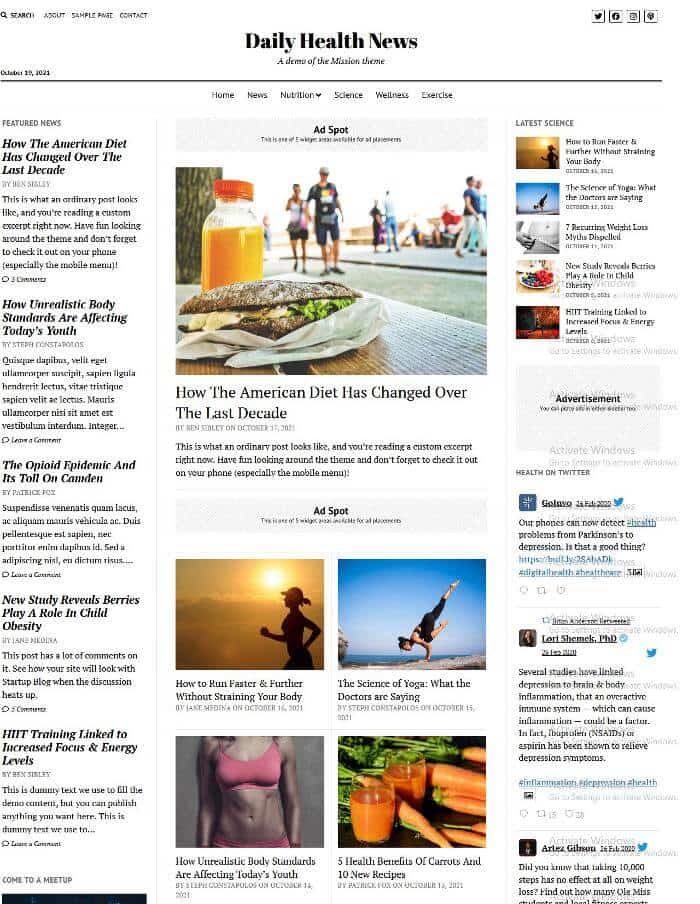A screenshot of a daily health news homepage from October 20th, 2021, featuring a white background with multiple news stories and images arranged in a grid-like layout. Each story is accompanied by a rectangular image and a bold black title beneath it. The text appears too small to read clearly, making it difficult to discern the content of the individual stories. The overall appearance is crowded and challenging to navigate.